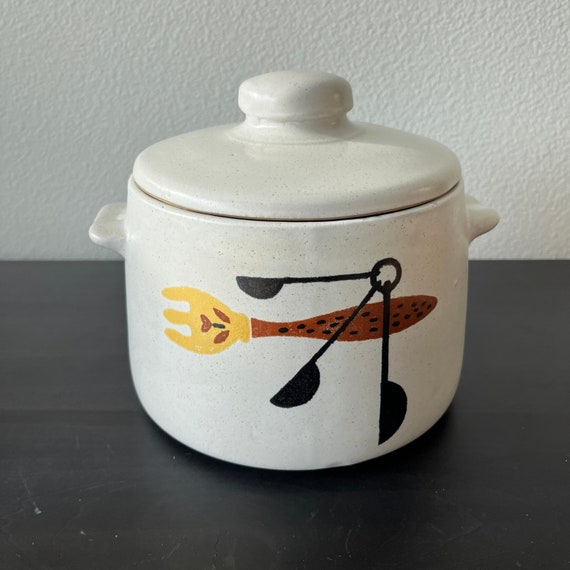This photograph captures a thick, off-white ceramic canister with a lid, featuring two short handles on either side. The lid sports a built-in, circular knob at its center. The canister sits on a dark wooden table, against a textured white wall, and is adorned with a colorful, painted fork on its front. The fork, positioned horizontally with its prongs pointing left, has a brown, black-speckled handle and an orange-gold pronged end with a distinct red mark. Laid over this vivid fork painting is a set of three black measuring spoons, clustered together on a ring located just above the fork's handle, adding a functional yet decorative layer to the scene.